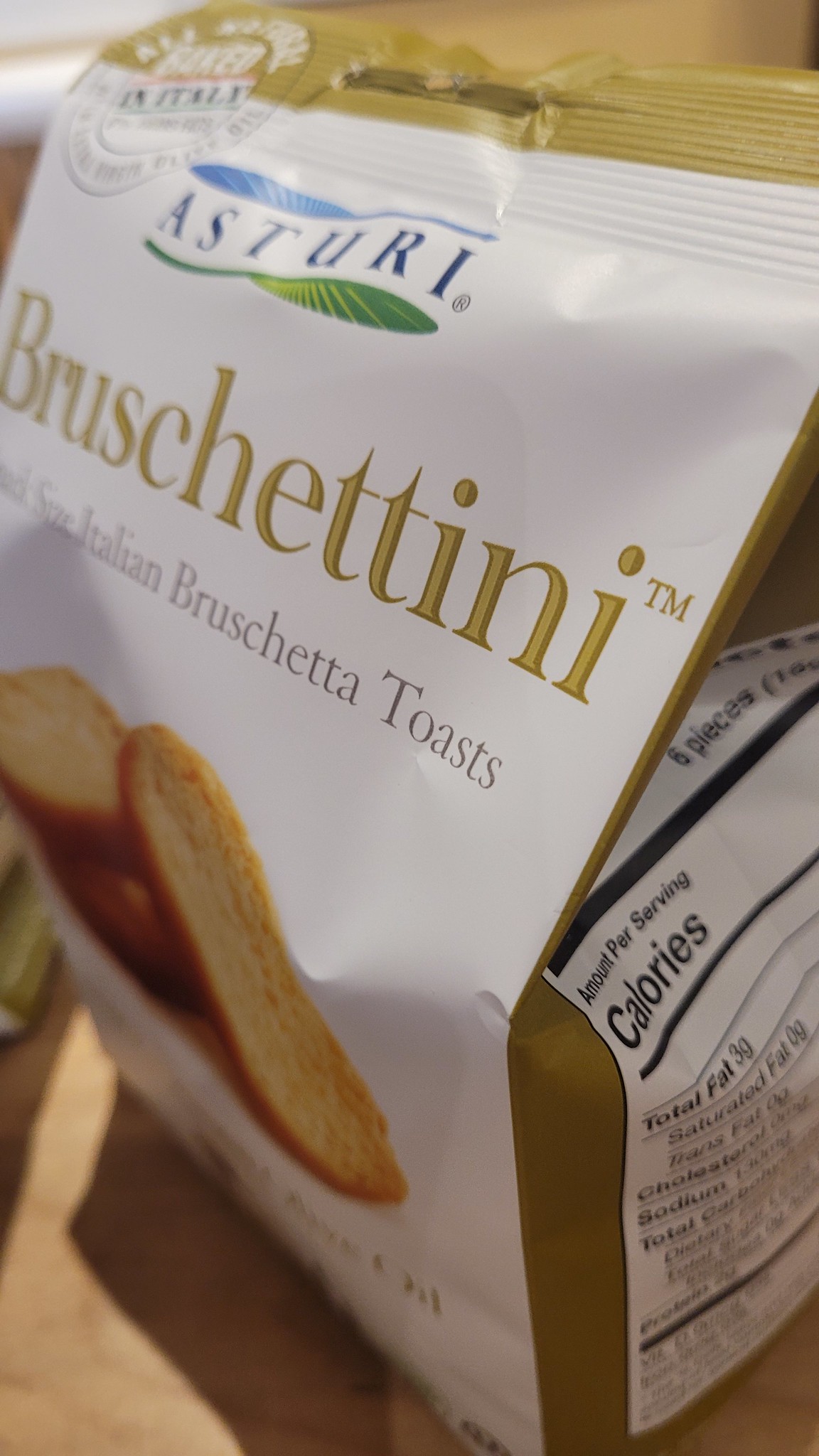The image features a colorful photograph of a bag of bruschettini made by the brand Ossituri. The word "bruschettini" is prominently displayed in elegant gold letters with a trademark symbol (™) at the end. Just above, the brand name "Ossituri" is adorned with a green leaf at the bottom and a blue leaf at the top. Off to the left, there is an indistinct circle with text that is hard to decipher. 

The main part of the bag is predominantly white with a brown edge. It features a tear-apart closure. Through a transparent section on the front, you can see the product inside—long, oval-shaped pieces of toasted Italian bruschetta. A partially visible section on the side of the bag includes some nutritional information, indicating that the total fat content is three grams per serving, although the rest of the details are difficult to read due to the bag being bent and cut off.